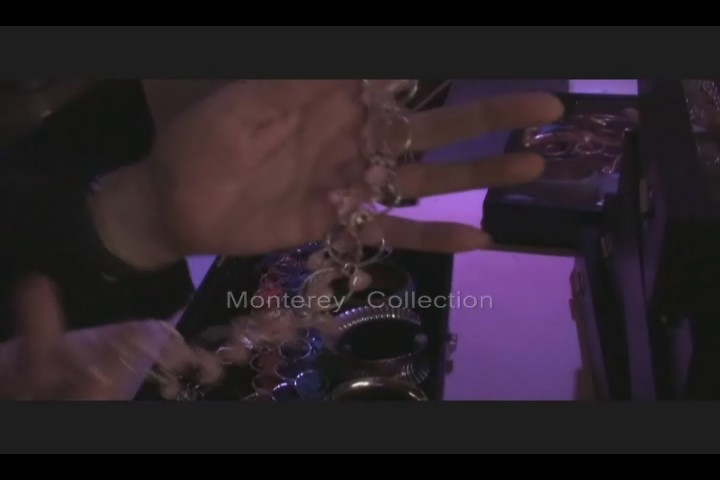In this rather dark and somewhat blurry image, there is a black rectangular border framing the entire scene. Inside the frame, a person's left hand, possibly female, is prominently displayed with the palm facing towards the viewer, showing traces of motion. The wrist is partially covered by a black outfit. The hand is holding up some intricate circular chain-link jewelry adorned with various colored gems such as red and blue. Beneath the hand, on what appears to be a mirrored surface, there is more jewelry and indistinct, fuzzy black containers that likely store these items. The words "Monterey Collection" are visible in white on the mirrored surface. The background has hints of purple, adding to the overall dark tone of the photograph.